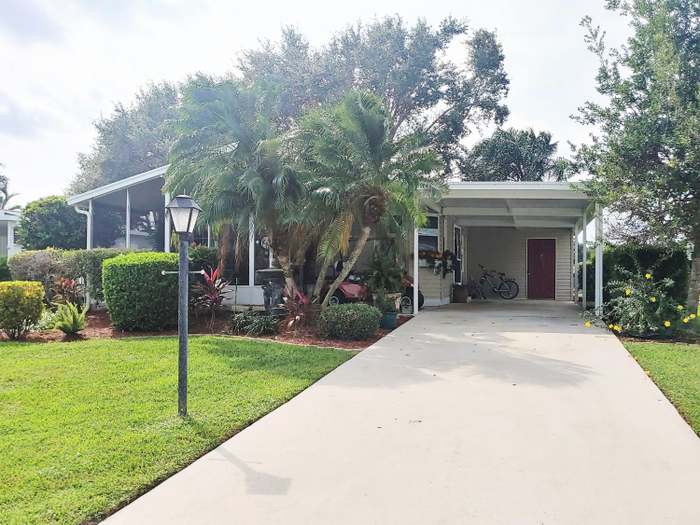This daytime photo captures the front of a residential house, taken from the perspective of the sidewalk looking down a long, light gray concrete driveway, which is offset to the right-hand side of the image. To the right of the driveway is a well-manicured green lawn adorned with large green hedges, palm trees, and a black lamppost with a glass lamp shade. The house features light tan horizontal siding and appears to be a mobile home or trailer park style. It is a single-story structure with a flat, pitched roof. 

At the end of the driveway, there is a red burgundy door underneath a white awning supported by a white post. A bicycle is parked in front of the door, and to the left of the door, there's a covered parking area where more details come into view. This area includes huge floor-to-ceiling windows, suggesting a covered porch or solarium, and a golf cart can be seen through the windows. In the background, large trees and wispy, white clouds in a bright sky complete the scene. Shrubs and more tropical trees line the front of the house, adding to the neat and tidy appearance of the property.